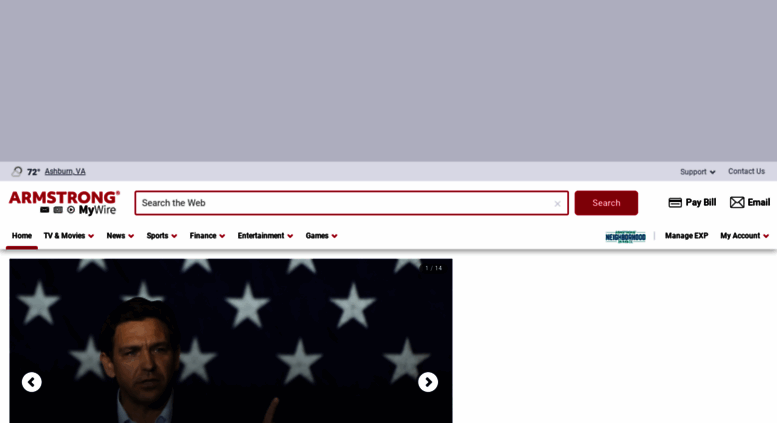Screenshot Description: 

The screenshot features a website interface with a predominantly white and red color scheme. At the top is a light purple field that spans the full width of the site, currently blank. Below this, there's a weather widget displaying a partly cloudy icon and the temperature "72" in Ashburn, Virginia. To the right of this widget, options for "Support" and "Contact Us" are available.

The next section shows the branding of the website: "Armstrong," in prominent red text, followed by "MyWire." Adjacent to this branding is a red-bordered search field labeled "Search the web," with a matching red search button to its right. Continuing to the right, there are two icons—a credit card icon with the text "Pay Bill" and an envelope icon labeled "Email."

Below this header, a navigation menu is present with several options: "Home" (highlighted with a red bar), "TV and Movies," "News," "Sports," "Finance," "Entertainment," and "Games." Each navigation item, except "Home," includes red down-arrow drop-down indicators.

The primary content area of the screenshot displays an image of Ron DeSantis, the Governor of Florida, standing in front of an American flag. The blue field with white stars of the flag is clearly visible. To the right of the image are forward and back buttons for navigating through a photo slideshow. The remainder of the page below this area is a blank white field.

This detailed description provides a clear, comprehensive understanding of the website's layout and content as seen in the screenshot.